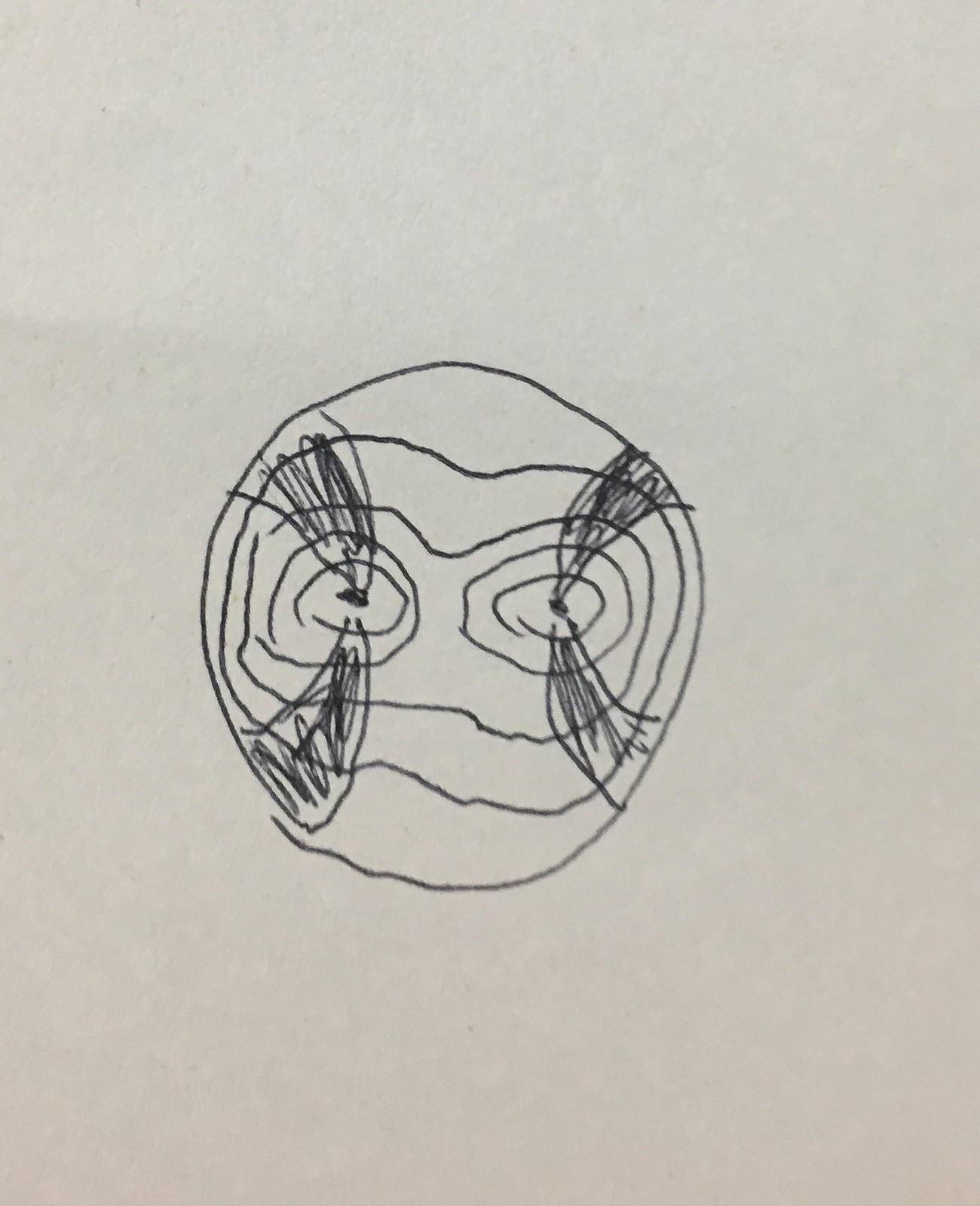This detailed photograph captures a white piece of paper with a singular, subtle wrinkle positioned slightly above the center on the left side. The delicate crease casts a faint shadow, discernible only to a keen observer. Central to the paper's composition is an intricate black pen drawing. Dominating the center is a large circle. Inside this primary circle, there is a smaller, mask-shaped circle, which is itself nested within another circle. Flanking this central composition are two additional circles, each containing two more circles within them. At the heart of these nested circles are two black dots. Emanating from the upper and lower edges of these dots are clusters of black, scribbled triangles, adding an abstract and intriguing element to the artwork.